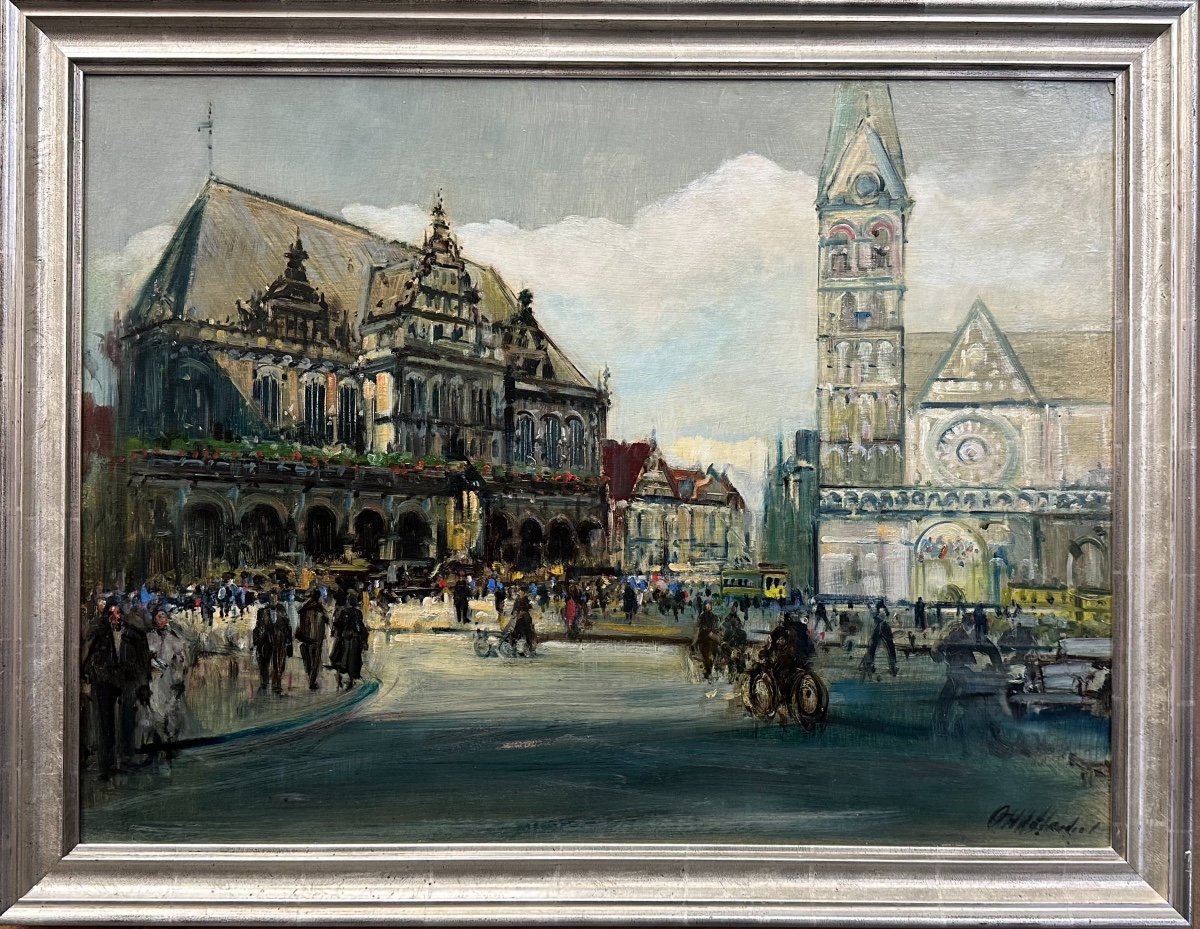This captivating oil painting, encased in a grayish silver metallic frame, depicts a bustling European city street, rich with historical architecture. Dominating the left side of the artwork is a majestic, gothic-style building featuring a steeple-topped roof and angular pointed rooms, rendered in dark brown and gray tones. Adjacent to it, toward the right, is a significant tower coupled with an elegant structure crowned by an angled brown roof.

In the foreground, a diverse crowd traverses the sidewalks and street; some are on foot while others ride bicycles, including a few on horseback. The presence of a yellow school bus among the figures subtly anchors the scene in a more modern time frame despite the old-world ambiance. Adding to the layered imagery, plants adorn a second-floor balcony of the left building, and further back, glimpses of houses with red roofs enhance the cityscape.

The street scene is lively with numerous people, predominantly clad in black, engaging in their daily routines. The overcast, cloudy sky, with hues of gray and fluffy white clouds mingling with patches of blue, sets a somewhat somber yet dynamic atmosphere. This intricate work of art is gracefully signed by the artist in the lower right corner, a testament to its intricate and thoughtful creation.